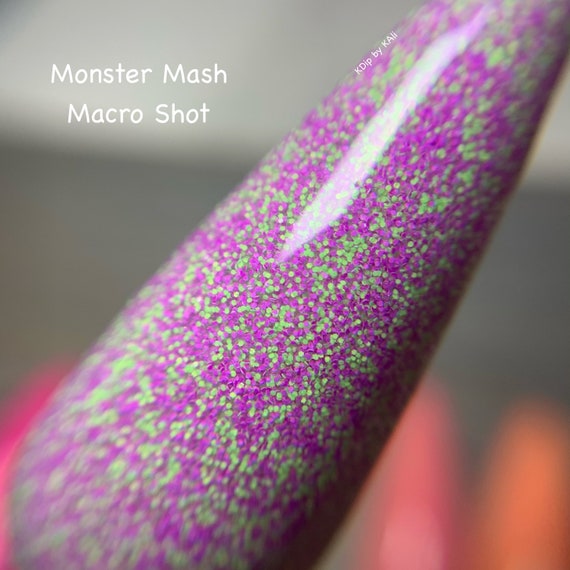This image is a square-cropped, extreme close-up macro shot of a woman's nail, shown from the upper right corner to the bottom left corner. The glossy nail is adorned with a striking fuchsia and green glitter flecked design, incorporating micro beads or round shapes in green and purple hues. A specular highlight creates a rectangular white reflection on the nail's surface. Overlaid on a grey background in the upper left corner are two lines of white text in a Comic Sans font, reading "Monster Mash Macro Shot." Additionally, a small watermark towards the upper right quadrant declares "K. K. Dip by Kali." The background appears blurry, showcasing grey at the top with a gradient to pink and orange at the bottom, enhancing the prominence of the nail art.